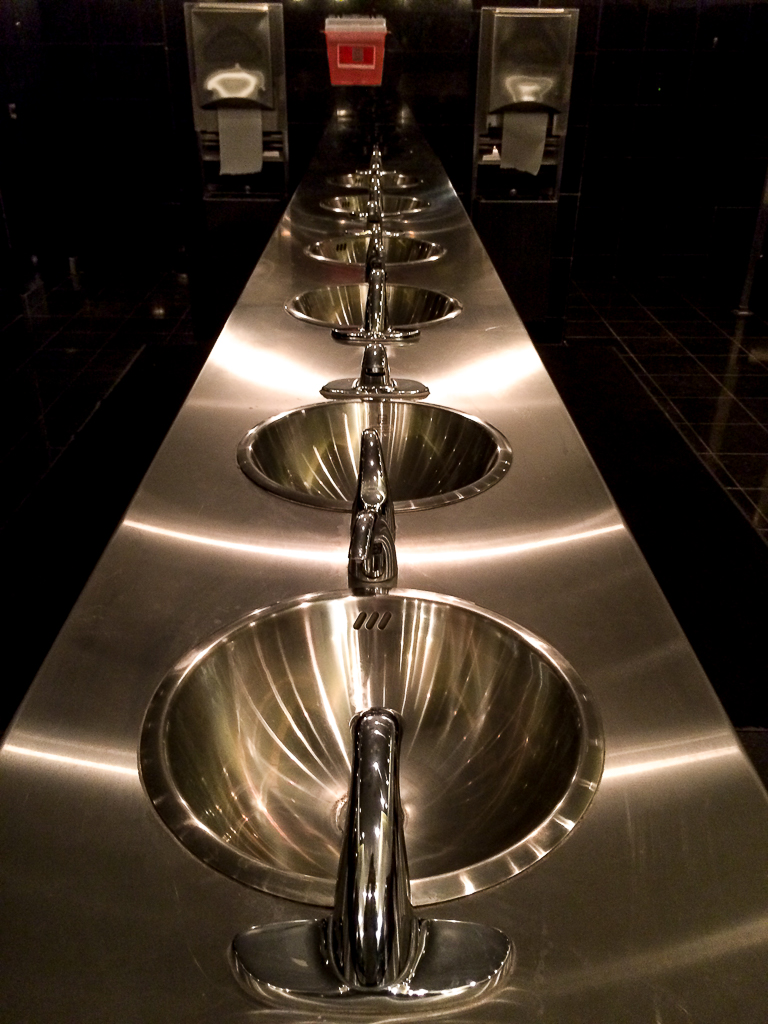This is a detailed photograph of a long row of five shiny stainless steel sinks, situated in a dark-tiled public restroom or facility. The perspective is from the end of the row, looking towards a wall mounted with two stainless steel dispensers on either side, dispensing thin rolls of what might be paper towels for hand drying. Between the dispensers, there is a red box-like item mounted on the wall, which could potentially be a soap dispenser or a hazardous material container. Each sink, characterized by its shiny metal bowl and faucets, reflects the overhead lighting, which casts linear reflections across the surface. The setup suggests a place where multiple people can wash their hands simultaneously, with the sinks and faucets uniformly aligned along the stainless steel counter.